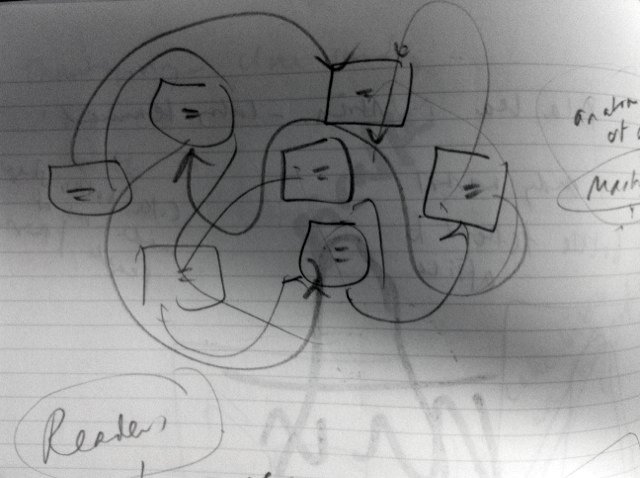This image is a detailed drawing on notebook paper in an indoor setting. In the bottom left corner, the word "READERS" is written and circled, spelled out in capital letters, R-E-A-D-E-R-S. The drawing features seven squares connected by arrows in a crisscross, snake-like pattern, with each square containing an equal sign. On the outer right side, there is a phrase that reads "an atom of" followed by a circular shape labeled "mash." There is also bleed-through from the reverse side of the paper, showing a black X, some circles, and letters.